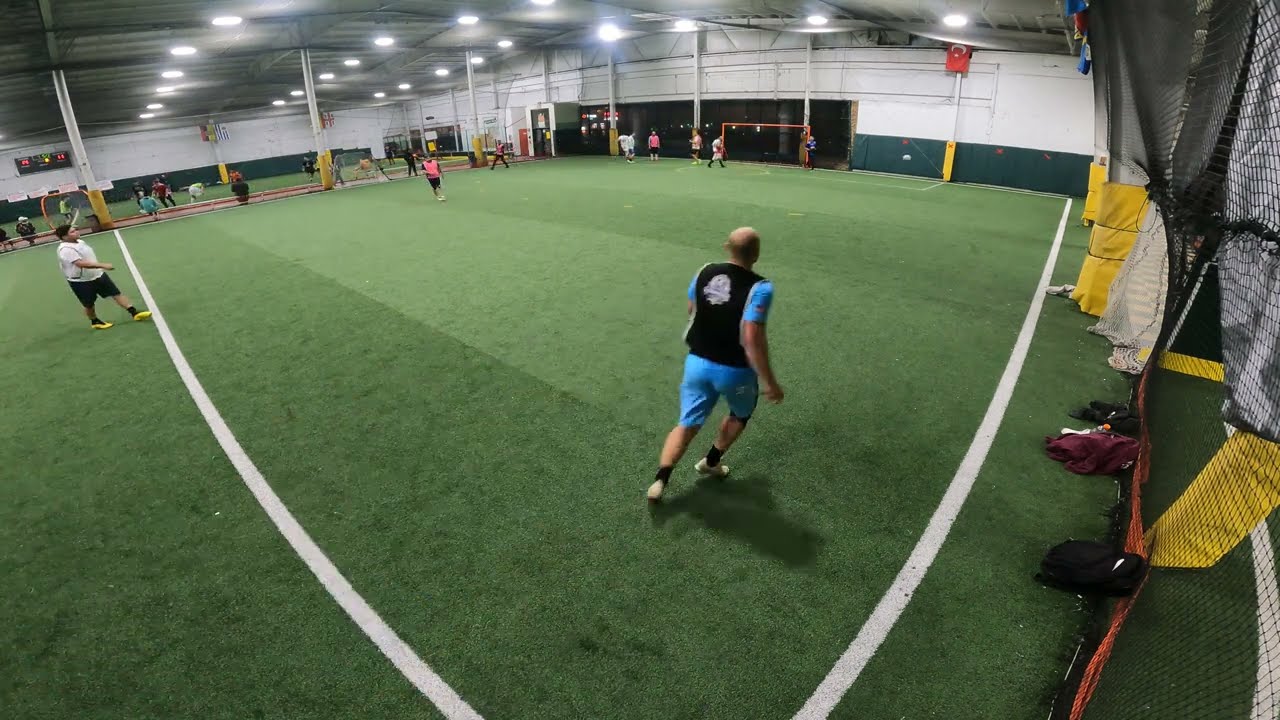The image depicts an indoor sports field housed within a large metal building characterized by a high ceiling supported by white columns with yellow padding at their bases. The ground is covered with green astroturf featuring distinct white boundary lines arranged in a square formation. In the center of the field, a balding man wearing blue shorts, black socks, and a blue and black top is running towards the right. To the upper left, there is a heavier-set individual in yellow sneakers, black shorts, and a white t-shirt. Scattered throughout the background, other people are walking and mingling, suggesting ongoing activities. A soccer goal is visible in the distance. The right side of the image features vertical netting from floor to ceiling, and some clothing appears to be discarded on the floor. The walls are painted white on the upper portion and navy blue at the bottom. From the ceiling, numerous spotlights cast a white light illuminating the field, resembling a warehouse environment.